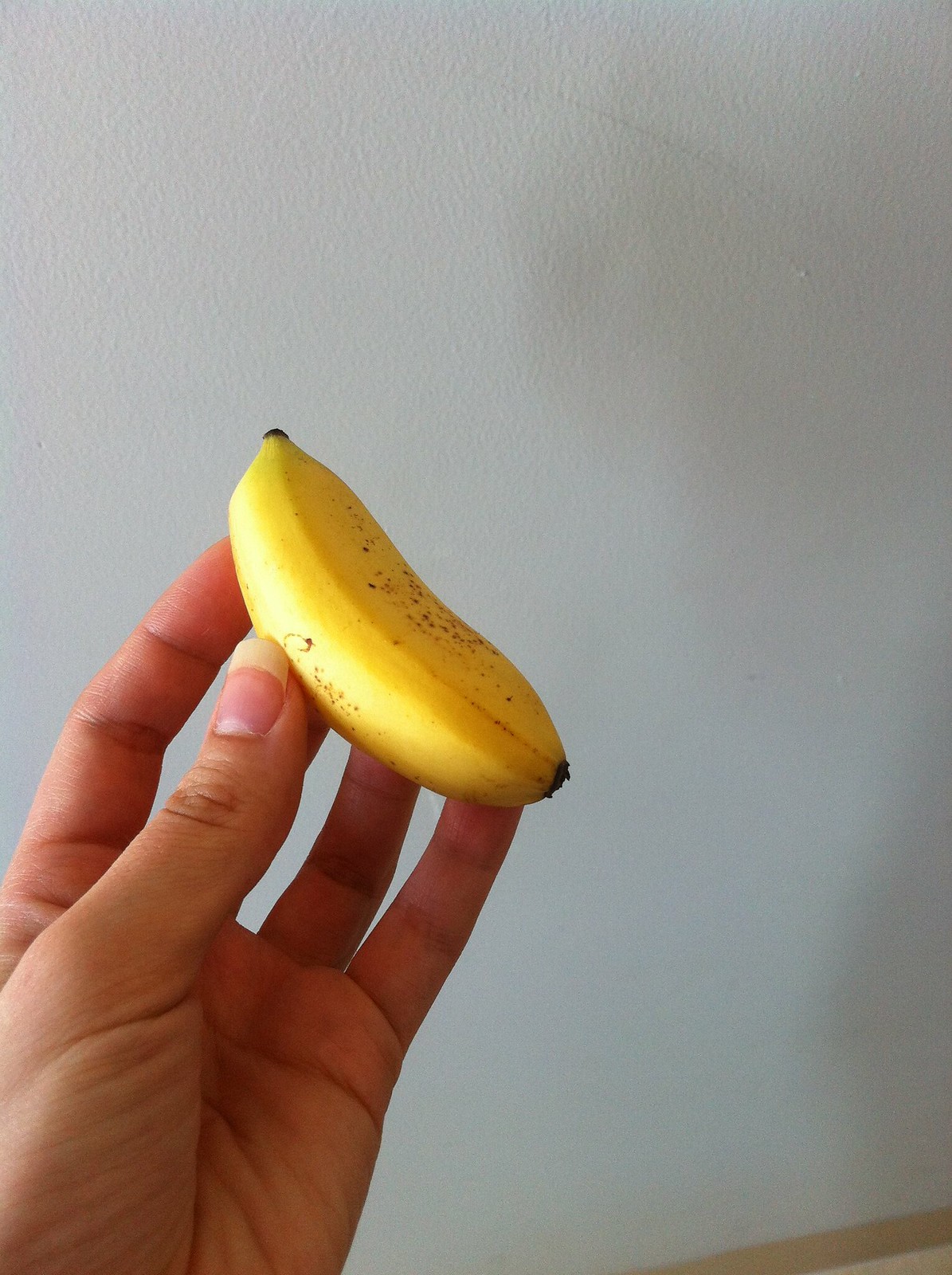In the image, a miniature banana rests in a hand, which belongs to a white person and is visible from the wrist. The hand, notable for its well-maintained fingernails, cradles the tiny banana between the thumb and four fingers, with the pinky finger slightly protruding. The banana, approximately two inches long, exhibits signs of aging and features a lacquering stamp as well as small, round spots on both its top and bottom halves. A light source casts a yellow glare along the side of the banana, highlighting its slightly worn surface. The background is predominantly white, albeit with a subtle shadowy gradient. In the left corner, part of a round strip is visible, possibly where a table intersects with the wall, adding a hint of spatial context. A deeper shadow lines the right side of the image, contrasting with the illuminated left side.